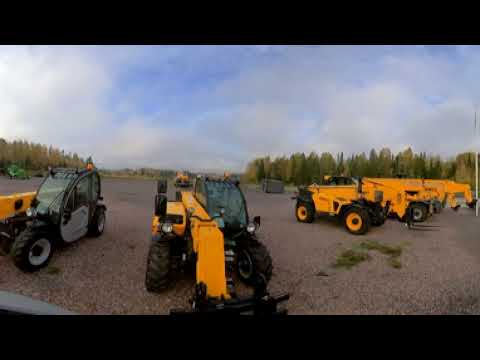In this outdoor image, a line of yellow and black heavy-duty construction vehicles stands out against a gravel and asphalt clearing. The equipment includes a variety of vehicles, some equipped with front scoops and arms, while others resemble small one-seater cars with crane or forklift attachments. The ground is a mix of rocks, gravel, and patches of small grass. A noteworthy gray and black tractor with a yellow arm is positioned to the left. Background features include densely packed, tall trees, with a slight clearing in the center that still retains some greenery. Above, the sky is mostly blue with scattered white and gray clouds. The setting creates a typical construction site atmosphere surrounded by natural elements.